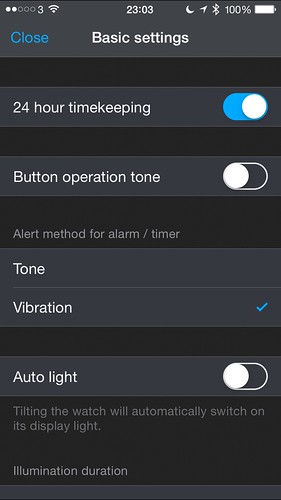This image is a screenshot taken from a mobile device, featuring a user interface with a dark gray and black background. The top section has a dark gray background with a variety of icons positioned in the left and right-hand corners. Centrally located at the top, the time is displayed as 23:03 with the battery status indicating a full 100% charge. To the far left of this bar, the word "CLOSE" is presented in blue, while centered prominently is the label "BASIC SETTINGS" in white text.

The main content area below is divided into different sections, each enclosed in separate boxes aligned vertically. The first section is labeled "24-hour timekeeping," accompanied by a slider that is colored white and blue, indicating that this option is turned on. The next section is titled "BUTTON OPERATION TONE," with an adjacent slider where the circle slider is positioned to the left, signifying that this feature is turned off.

Following this, in smaller text, is the label "ALERT METHOD FOR ALARM / TIMER," with two options listed below it: "TONE" and "VIBRATION." A small blue checkmark is shown next to "VIBRATION," indicating that vibration is the selected alert method.

Further down, another section labeled "AUTOLIGHT" features a similar slider as the previous ones. Here, the circle is also positioned to the left, depicted solely in white, indicating this feature is turned off. Beneath this, detailed text explains the feature: "TILTING THE WATCH WILL AUTOMATICALLY SWITCH ON ITS DISPLAY LIGHT."

At the very bottom left-hand corner of the interface, the text "ILLUMINATION DURATION" is displayed, concluding the detailed description of the settings presented in the screenshot.